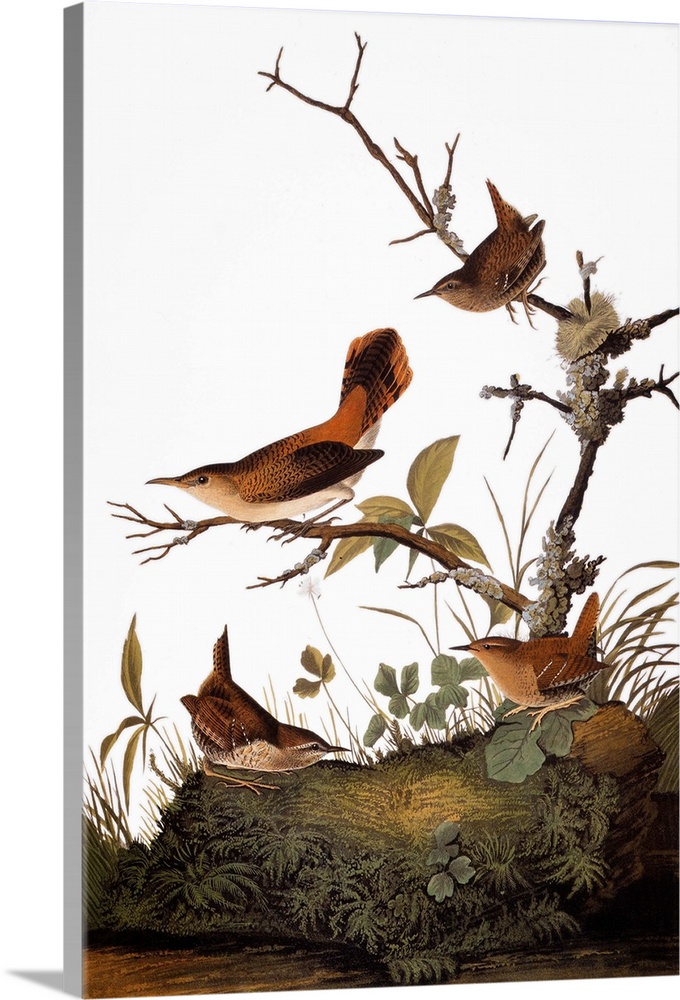The image is of a hand-drawn, detailed painting on a canvas with dimensional texture. The painting features a serene natural scene with a white background, showcasing four birds perched on branches and a moss-covered log. The composition includes a lower branch from which two smaller twigs extend; one houses a red bird with a dark brown center, white underside, and wings tipped in brown, its tail fanned up, and facing outward. The upper twig supports a smaller bird, similarly attentive, with brown feathers and darker brown accents. 

On the ground log, two birds face each other: the left one, crouched with a darker brown body and white belly, and the right one, which has a lighter brown chest and a darker back. Both the log and branches are adorned with greenery, including leaves, grass, and hints of moss, contributing to the lush, earthy ambiance. The birds have long, pointy beaks and legs, grasping the twigs confidently. The scene is enhanced by the presence of three-leaf and four-leaf clovers, adding a touch of whimsy to the natural setting. 

Despite its intricate detailing and neutral color palette, the painting does not bear the signature of its artist, inviting curiosity about its origin. This piece could easily be envisioned as part of an online art sale or displayed in a museum gallery, admired for its meticulous depiction of birds in a tranquil, natural habitat.